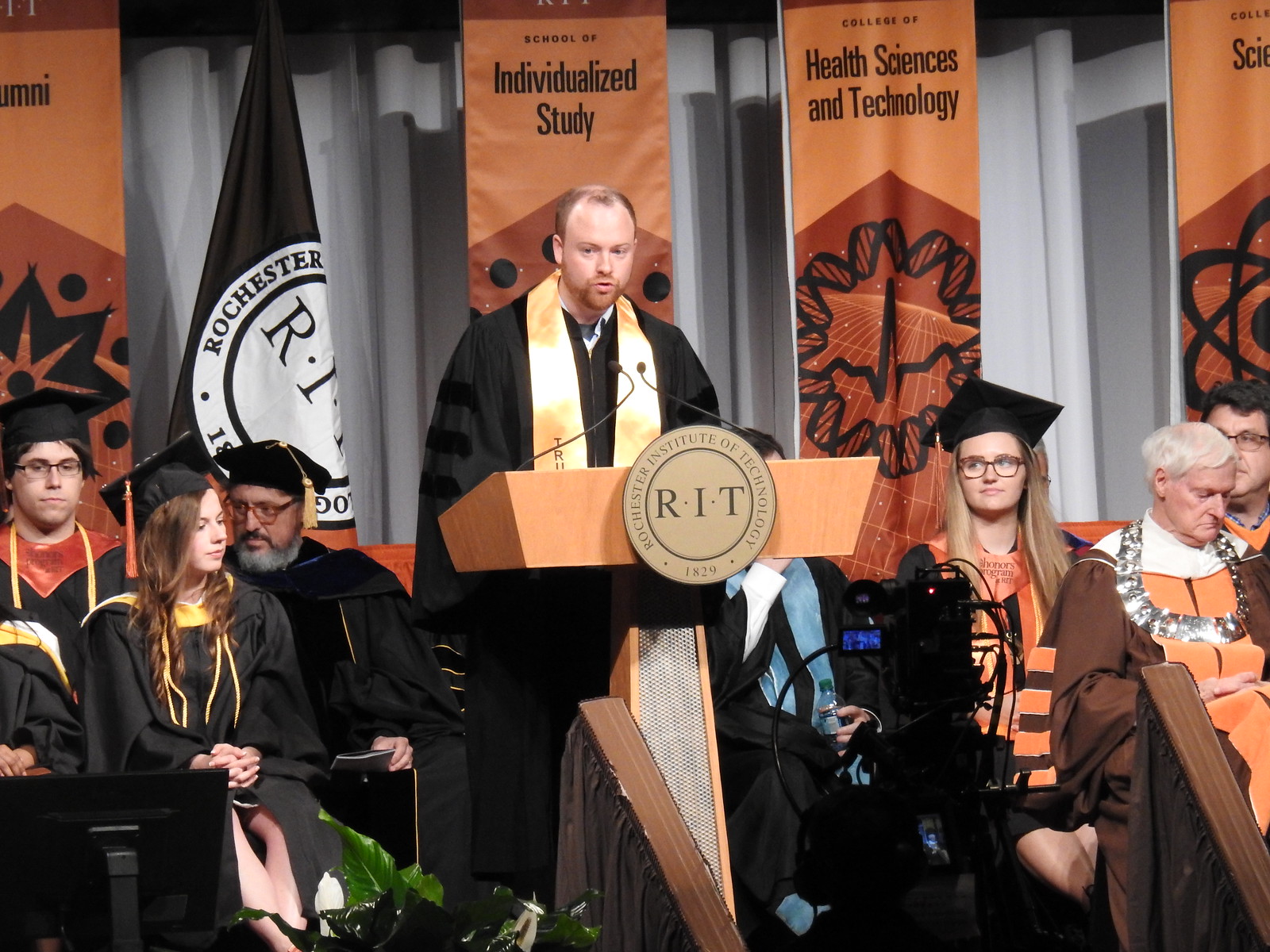The image depicts a graduation ceremony at the Rochester Institute of Technology (RIT). A white man with light brown hair, a sparse beard of the same color, and possibly in his 30s or 40s, stands at a brown-orange podium adorned with the text "Rochester Institute of Technology 1829" along with the acronym "RIT" on a gold-colored circular emblem. He is wearing a black graduation gown and a golden stole. In front of him are microphones. Seated behind him on stage are other graduates, some dressed in black gowns with black caps, while others wear brown gowns. The setting features a gray curtain backdrop with orange signs indicating "School of Individualized Study" and "College of Health Sciences and Technology." The audience comprises mainly white individuals appearing to be in their 20s and 30s, with a few older attendees present. A brown RIT flag is visible on the left side of the image.